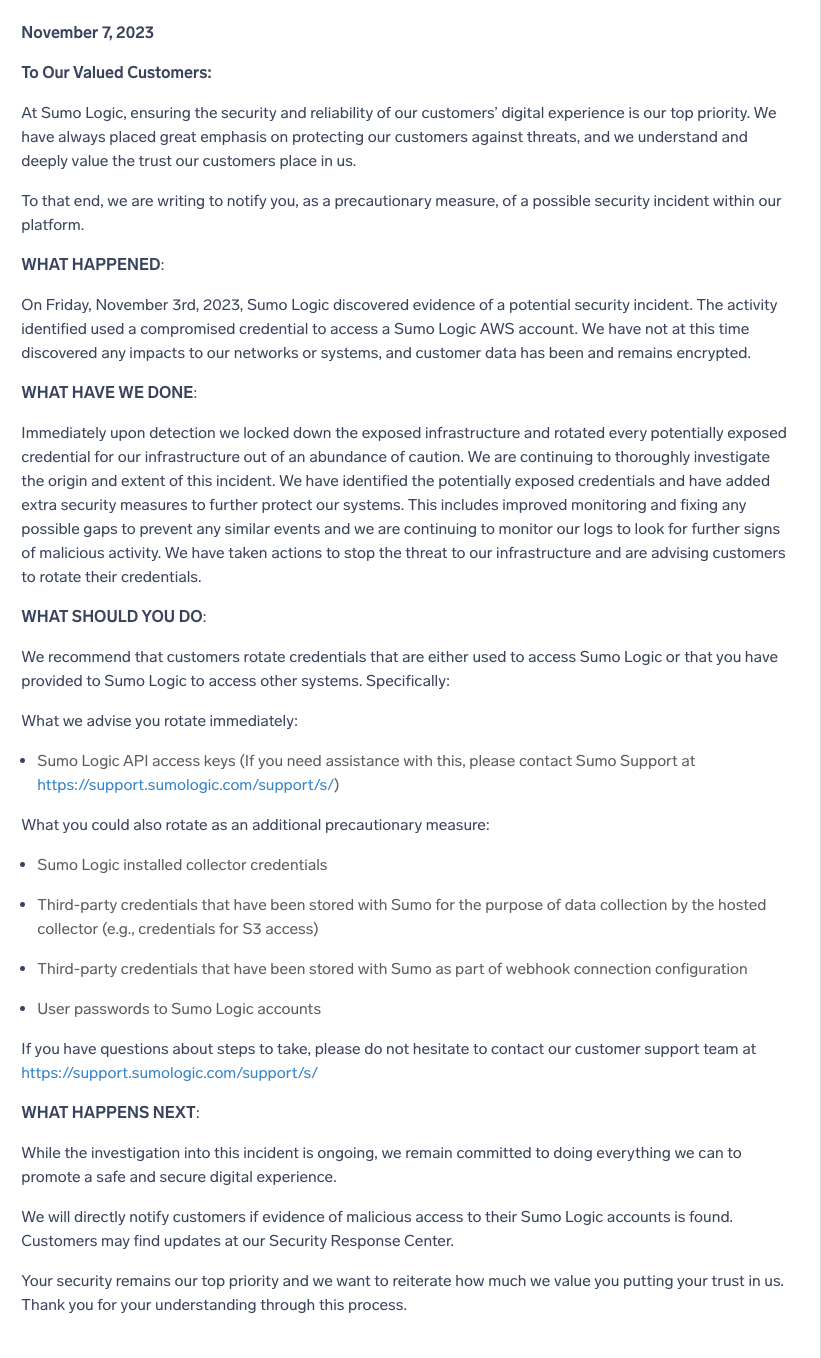**Detailed Caption:**

On November 7th, 2023, Sumo Logic issued a notification to its existing customers detailing a precautionary measure regarding a potential security incident on their platform. The announcement, titled "To Our Valued Customers," outlines a brief overview of the event, indicating that they have discovered evidence of a possible security breach.

The communication elaborates on the actions taken to mitigate the threat, including the immediate lockdown of the exposed infrastructure and the rotation of all potentially compromised credentials. Sumo Logic provides a comprehensive list of steps they have taken to fortify their security posture and advises customers to take similar precautions.

Customers are urged to rotate credentials associated with Sumo Logic or those provided to Sumo Logic for accessing external systems. A meticulous list of specific tasks for customers to follow is included to ensure the highest levels of security.

The notification concludes with a reassurance that Sumo Logic is actively investigating the incident and remains dedicated to maintaining a secure digital environment. Customers are promised direct communication if any malicious access to their data is confirmed.